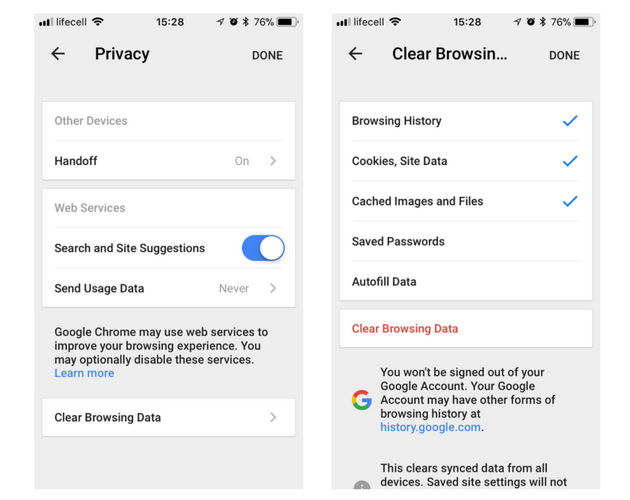The image consists of two screenshots placed side-by-side.

### Left Screenshot:
- **Top Status Bar**: 
  - Signal Strength: Three bars
  - Label: "Lifestyle"
  - Connectivity Indicators: Full Wi-Fi signal
  - Time: "1528"
  - Other Indicators: Directional arrow, alarm clock, Bluetooth icon, and 76% battery level.
- **Main Interface**: 
  - Background Color: Gray
  - **Top Row**:
    - Left: Black arrow pointing left
    - Center: Bold black text saying "Privacy"
    - Right: Capitalized black text "Done" in smaller font
  - **Settings Section**: 
    - **White Box 1**:
      - Top-left Label: "Other Devices" in gray text
      - Divider: Gray line
      - Setting: "Handoff"
        - Status: "On" (in gray text) with a right arrow
    - **Gray Divider**: 
    - **White Box 2**:
      - Section Title: "Web Services" in gray text
      - Divider: Gray line
      - Setting: "Search and Cite Suggestions"
        - Status: Turned on (indicated by a blue slider button)
      - Divider: Gray line
      - Setting: "Send Usage Data"
        - Status: "Never" (in gray text) with a right arrow
    - **Additional Information**:
      - Text: "Google Chrome may use web services to improve your browsing experience. You may optionally disable these services."
      - Link: "Learn More" in blue text
    - **White Box 3**:
      - Setting: "Clear Browsing Data" with a right arrow

### Right Screenshot:
- **Top Status Bar**: Identical to the left screenshot 
  - Signal Strength: Three bars
  - Label: "LifeCell"
  - Connectivity Indicators: Full Wi-Fi signal
  - Time: "1528"
  - Other Indicators: Directional arrow, alarm clock, Bluetooth icon, and 76% battery level.
- **Main Interface**: 
  - Background Color: Gray
  - **Top Text**:
    - Left: Black arrow pointing left
    - Center: Bold black text saying “Clear Browsing...”
    - Right: Capitalized black text "Done" in smaller font
  - **Settings Section**:
    - **White Box 1**:
      - Setting: "Browsing History"
        - Status: Blue check
      - Divider: Gray line
      - Setting: "Cookies, Site Data"
        - Status: Blue check
      - Divider: Gray line
      - Setting: "Cached Images and Files"
        - Status: Blue check
      - Setting: "Save Passwords"
      - Setting: "Autofill Data"
      - Divider: Thin gray stripe
    - **White Box 2**:
      - Button: "Clear Browsing Data" in red text
      - Additional Information: 
        - "You won't be signed out of your Google account. Your Google account may have other forms of browsing history at"
        - Link: "history.google.com" in blue text
        - "This clears sync data from all devices. Save Site Settings, Will Not"

This detailed caption provides a thorough description of both screenshots, encapsulating all visible elements and their respective statuses or labels.